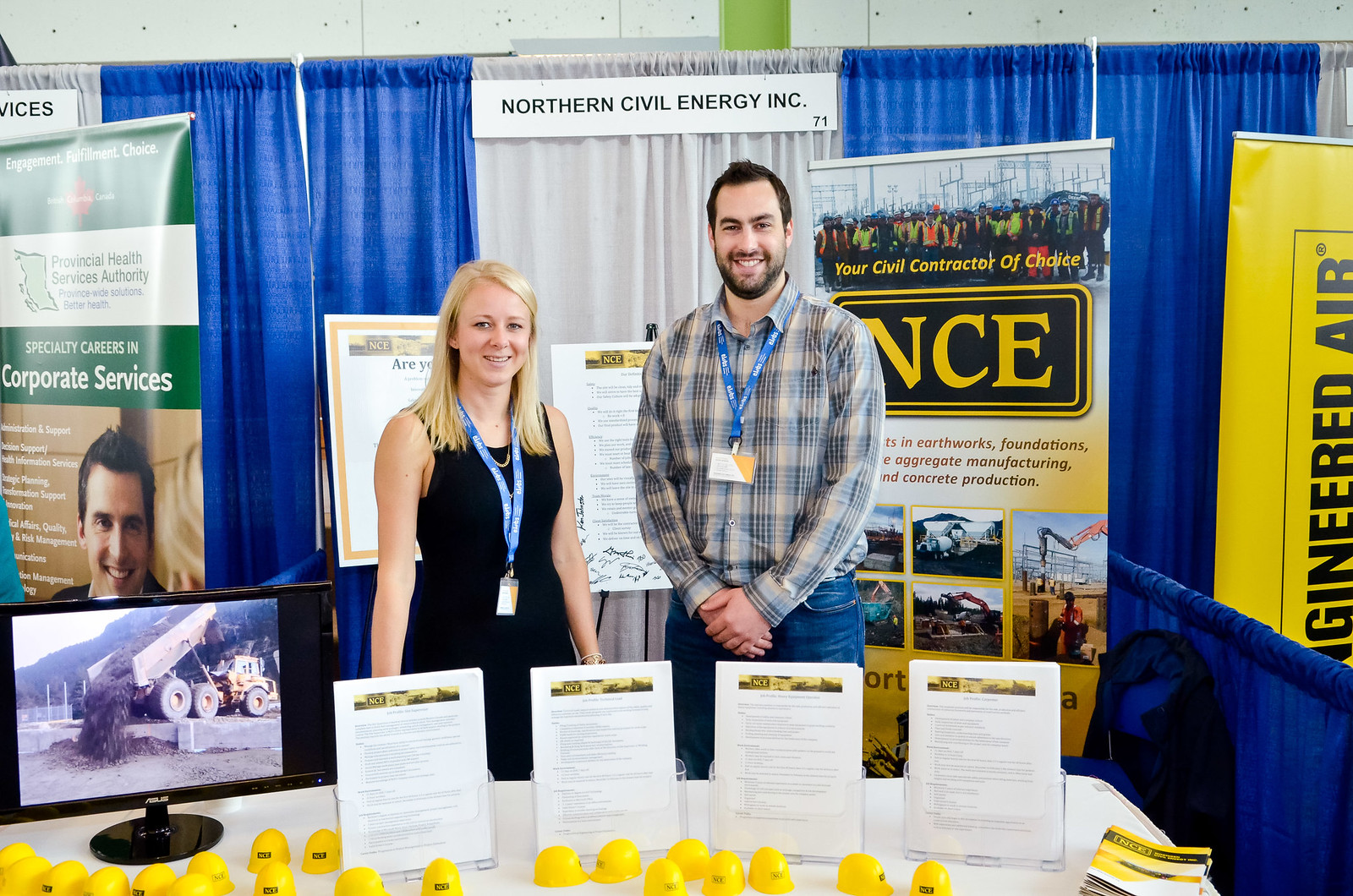At a bustling conference booth or hiring event for Northern Civil Energy, Inc., a young blonde woman in a black dress and a plaid-clad man with dark hair and a beard stand ready to recruit. Both wear blue name badges and ID tags around their necks. Positioned behind a display table adorned with colorful pamphlets, flyers, and papers that detail the company’s offerings, they present an inviting array of materials including yellow construction hats. The booth prominently features signs declaring Northern Civil Energy as "Your Civil Contractor of Choice," specializing in "Earthworks, Foundations, Aggregate Manufacturing and Concrete Production, and Engineered Air." A TV monitor to the left showcases a massive dump truck emptying a load of dirt at a worksite, adding a dynamic visual to the setup. The scene captures the essence of a professional recruitment effort, emphasizing the company’s extensive services and career opportunities in civil contracting.